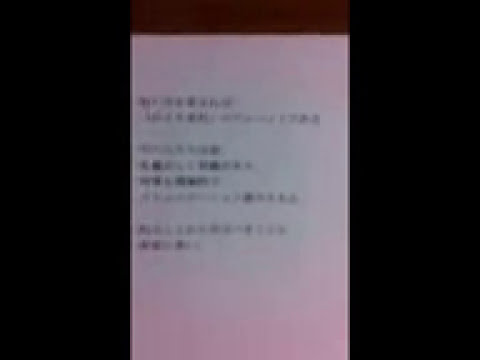The image features a very blurry piece of paper with black text that appears to be a receipt or notice, written in Asian characters that are indecipherable. The background of the photo is black, with a dark brown streak across the top. The paper itself is not simply white but appears to have a faded light pink hue, particularly at the top and bottom. The photo is vertically letterboxed, with the letterboxes being as prominent as the main image itself. There are approximately eight lines of text or numbers on the paper, but due to the extreme blurriness, the content remains unreadable.